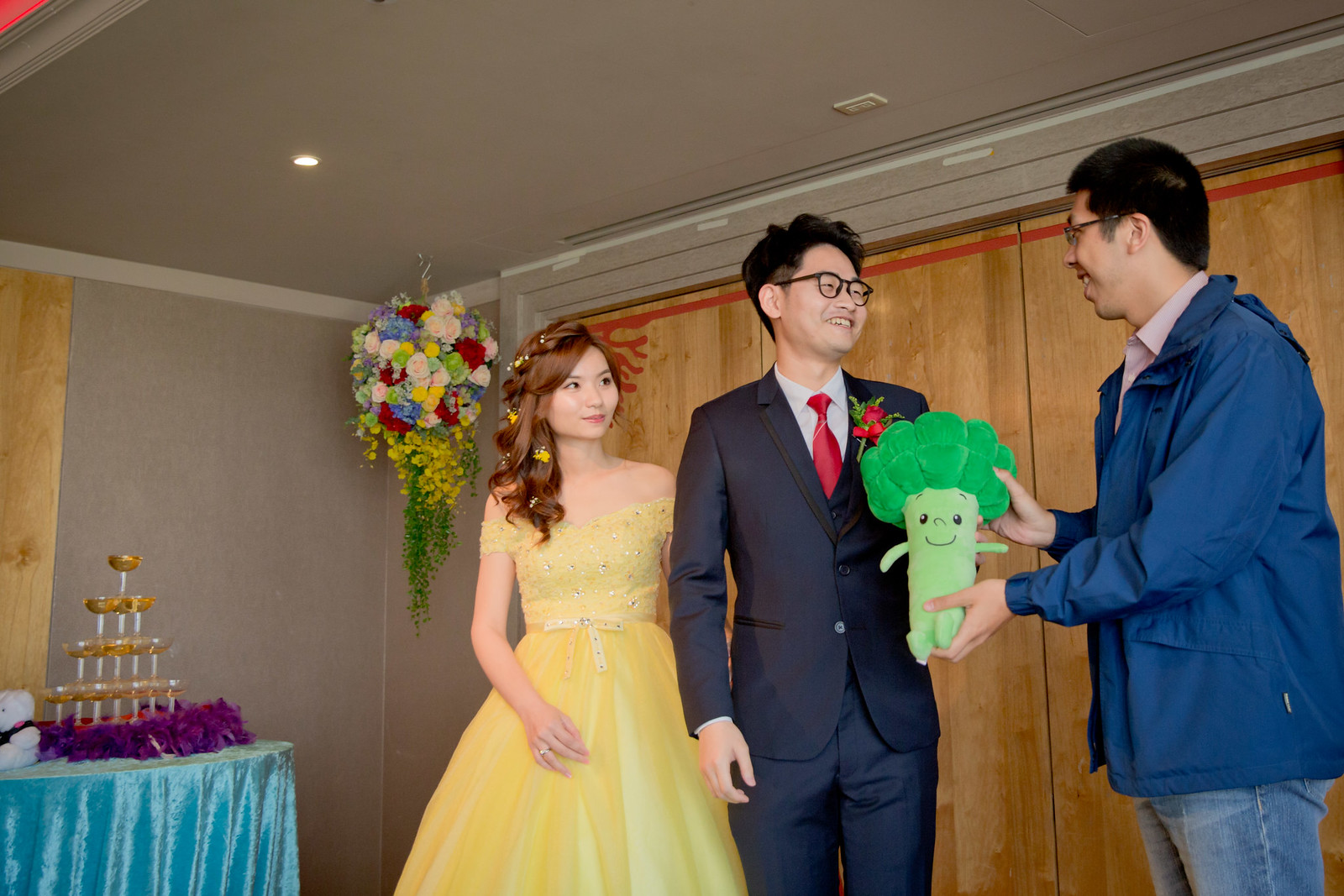This photograph captures a joyful celebration, likely a wedding or engagement in an Asian setting. The scene is set in a room with a backdrop of three light wooden doors. In the center-left, a woman, with dark reddish-brown hair adorned with yellow flowers, is wearing an elegant yellow dress with a poofy tulle skirt. She is flanked by two men. The man next to her is wearing a dark suit with a red tie and a red rose on his lapel, paired with glasses. To his right, another man, dressed in a blue jacket over a pink shirt and blue jeans, also with glasses, hands him a whimsical broccoli-shaped plush toy. Both men are smiling warmly.

In the background, there is a round table draped with a blue velvet tablecloth, adorned with a champagne tower and a small white teddy bear. Above them, a large bouquet of colorful flowers hangs from the ceiling, adding to the festive atmosphere. Everyone in the photograph exudes happiness, reflecting the celebratory nature of the occasion.